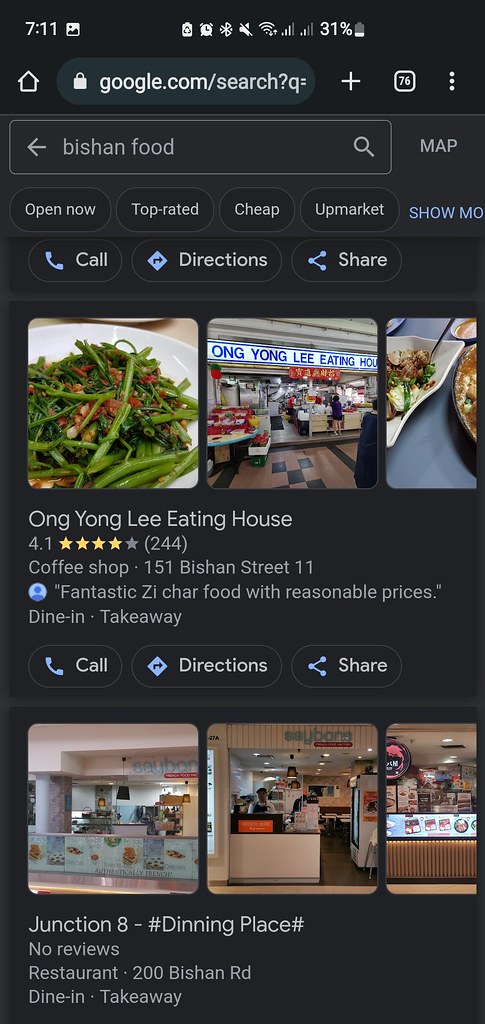This is a detailed, cleaned-up caption for the described image:

"A screenshot from a smartphone displaying the time as 7:11 AM. The status bar shows three signal bars on the left and two on the right, with the volume muted and 31% battery remaining. Below the status bar, the home icon, a lock icon, and the address bar (showing 'google.com/search?q=') are visible. The search query entered reads 'Bishan food.' The search results feature three thumbnails: one with string beans and red-tinted food, another depicting the interior of a restaurant with people in line, and a third showing a plate of rice with brown-colored dishes. Below the thumbnails, information is provided for 'Ong Yong Lee Eating House' which boasts a 4.1-star rating from 244 reviews. It is categorized as a coffee shop located at 151 Bishan Street 11, renowned for its fantastic Z-Char food, offering both dine-in and take-out options at reasonable prices."